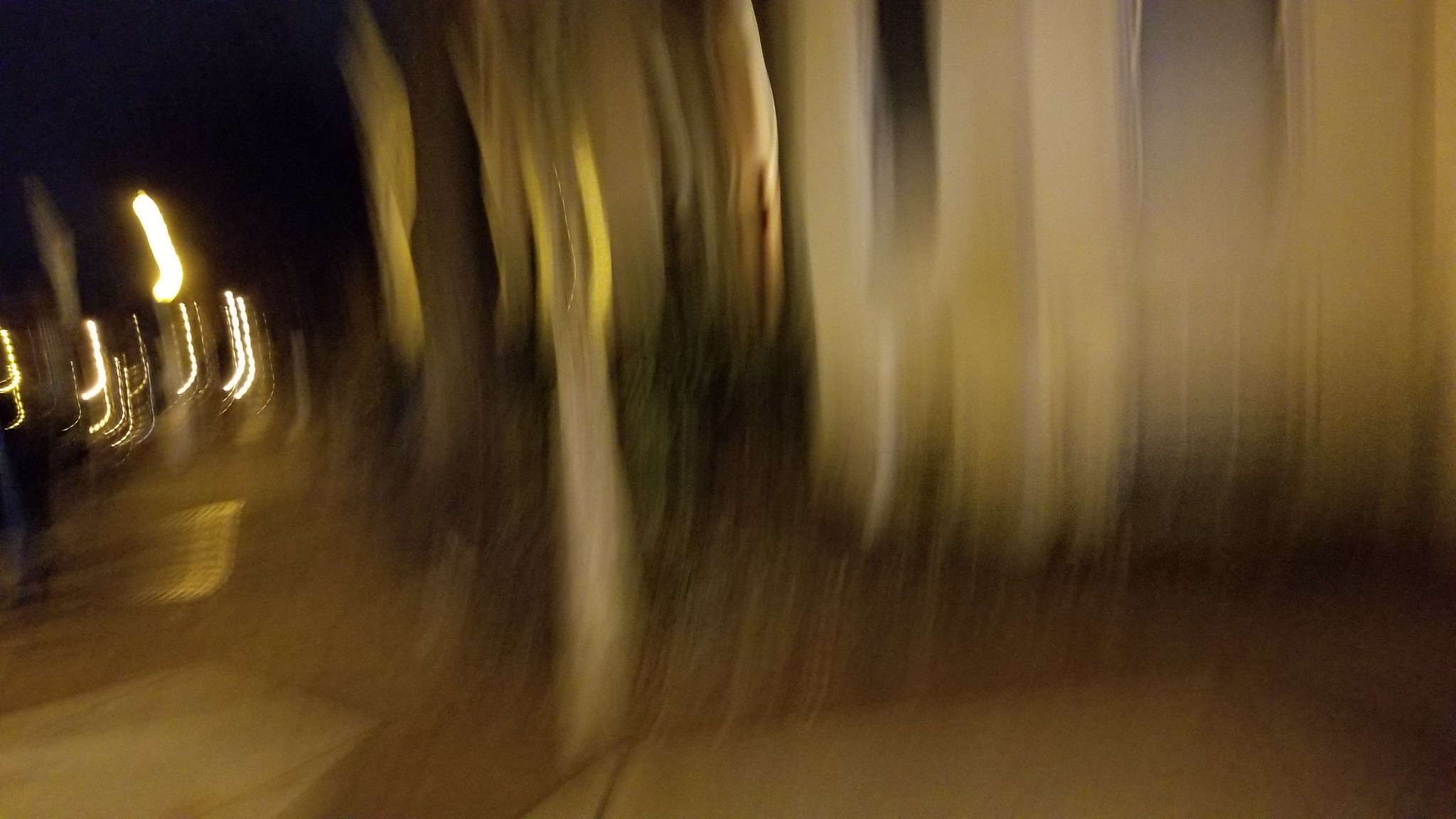This is an extremely blurry photo taken at nighttime, featuring a mix of beige, tan, brown, yellow, white, and black shades. The upper left-hand corner is black, likely indicating the night sky. On the left side, there are several indistinct lights, some of which seem to form a J-shape with a bright, curved section at the bottom. These lights are very bright, especially one that appears as the whitest, and others appear as dotted lines moving along this J-motion, possibly creating multiple shadows. Behind these lights, there might be the exterior of a building, potentially with windows and a porch area, or even lights outside a front door. In the middle, there are indistinguishable forms that look like brown and beige sticks with green behind them, suggesting they might be trees or bushes. Additionally, the blurred foreground features stripes of color that resemble fibers hanging down, reminiscent of a car wash but difficult to confirm due to the blurriness. Overall, the scene is hard to discern, but these elements hint at an outdoor setting with multiple light sources.